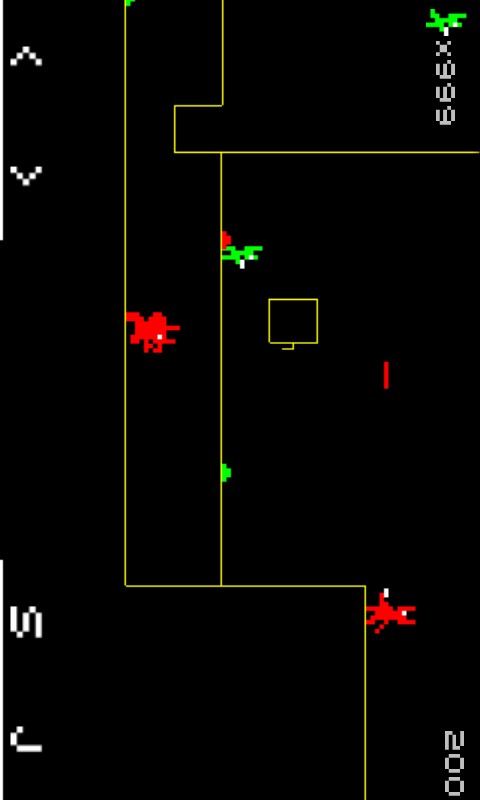This image is a screenshot from an old-school video game reminiscent of the 1980s, featuring a pixelated, retro style. The screen is oriented vertically, though the game appears to be designed for a horizontal landscape layout. The backdrop is predominantly black, creating a stark contrast with the vibrant pixelated elements. 

On the left side, there are up and down white arrows. Near the bottom left corner, the letters "SJ" are visible, albeit rotated, indicating the image itself may need to be flipped horizontally for proper viewing. In the bottom-right corner, the number "200" appears in grey.

The scene showcases various characters similar to those seen in classic games like Pac-Man or Space Invaders. Two red, pixelated creatures and one green character navigate the screen. The green character, seemingly armed with a small white gun that is just two pixels long, interacts with the environment, which consists of yellow lines serving as paths or obstacles. These lines form structures such as platforms to jump on, boxes, or gaps to navigate around.

Additionally, a green symbol displaying "x999" is visible, adding to the nostalgic interface reminiscent of early video games. The overall aesthetic and design evoke feelings of classic arcade gameplay, brought to life through a simplistic yet charming pixelated art style.